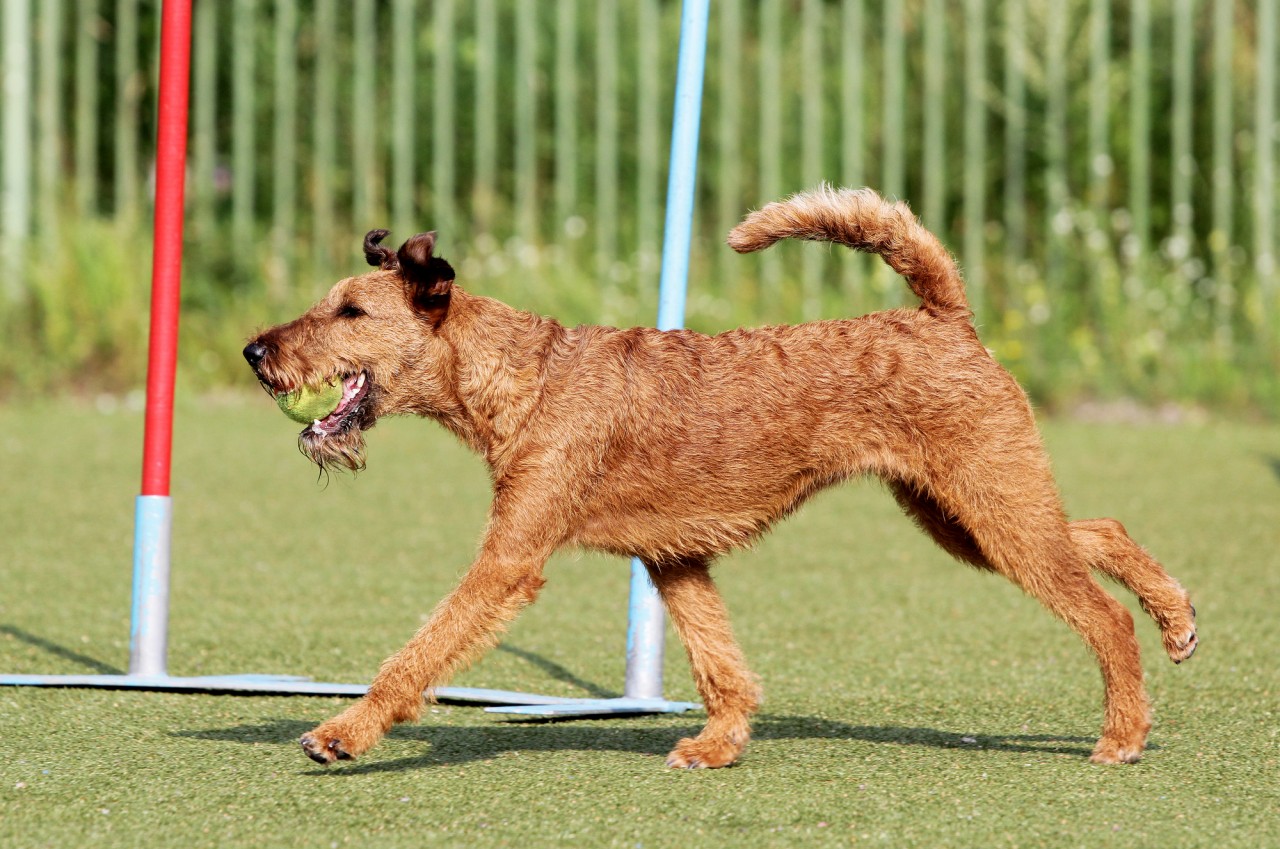This outdoor image features a medium-sized brown dog with black-tipped ears, exhibiting traits of both a doodle and possibly a spaniel or springer mix. The dog's coat is shaved short, revealing slight curls in its fur. Focused intently, the dog is captured mid-action with one leg extended forward, back leg up, and tail raised as it runs through an obstacle course. The scene is set in a grassy field, with low shrubs and a blurred fence comprising thin vertical rails in the background. Prominently visible are gray and orange obstacle poles, with a notable red pole intersecting the frame. The dog clutches a yellow tennis ball firmly in its mouth, poised for a successful run through the course. However, it eventually drops the ball after completing the challenges. The detailed background and dynamic posture of the dog emphasize the lively and competitive atmosphere of this event.